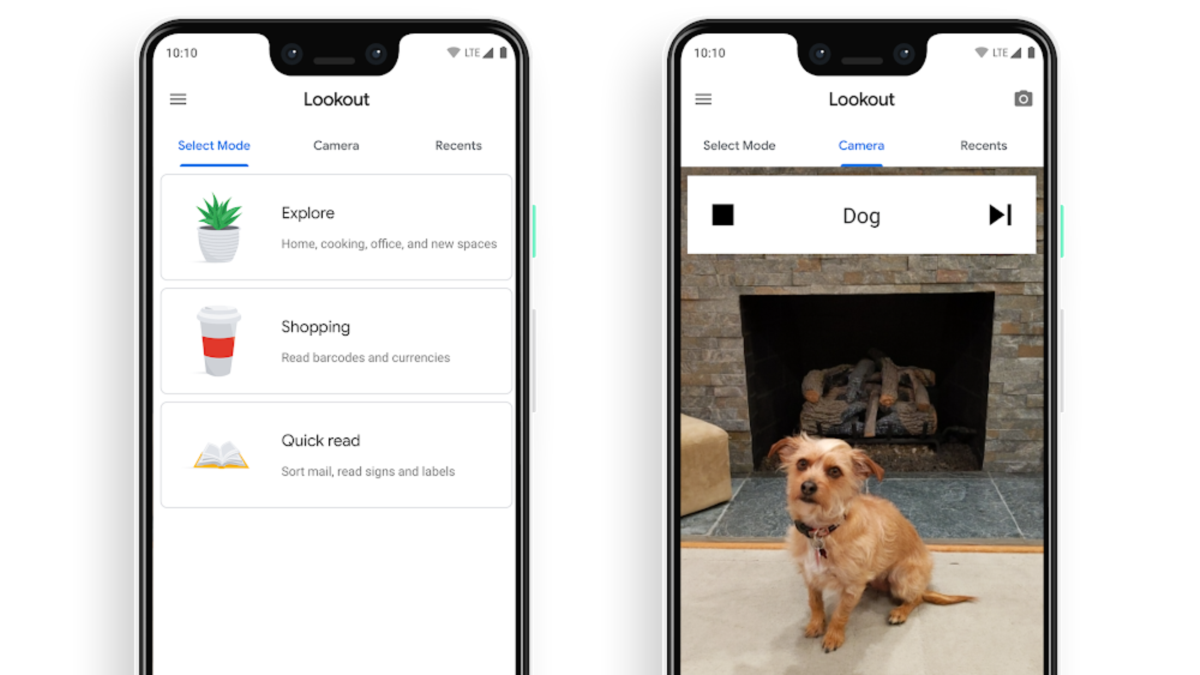The image showcases a dual-screen cell phone with detailed information displayed on both screens. 

**Left Screen:**
- The title at the top reads "Lookout" in black letters.
- The phone status indicators show it's connected to LTE, with a good battery life and a strong connection. The time displayed is 10:10 AM.
- Below the title "Lookout," the phrase "Select a mode" is written in blue, with options for "Camera" and "Recents" listed underneath.
- A highlighted option labeled "Explore" features a planter with greenery. Beneath it, various categories are listed: "Home," "Cooking," "Office," and "New Spaces."
- A section labeled "Shopping" displays an image of a white coffee cup with a red holder.
- Another section marked "Quick Read" shows a picture of a book and lists tasks like "Sort mail," "Read signs and labels."

**Right Screen:**
- It mirrors the left screen's layout with the title "Lookout" and the "Select mode" prompt, but here, "Camera" is underlined in blue, indicating it is the active mode.
- An actual photo of a dog sitting in front of a fireplace is displayed. The dog is on a cream-colored floor against a backdrop of green marble around what appears to be a faux fireplace. Part of a tan piece of furniture can be seen in the image's corner.